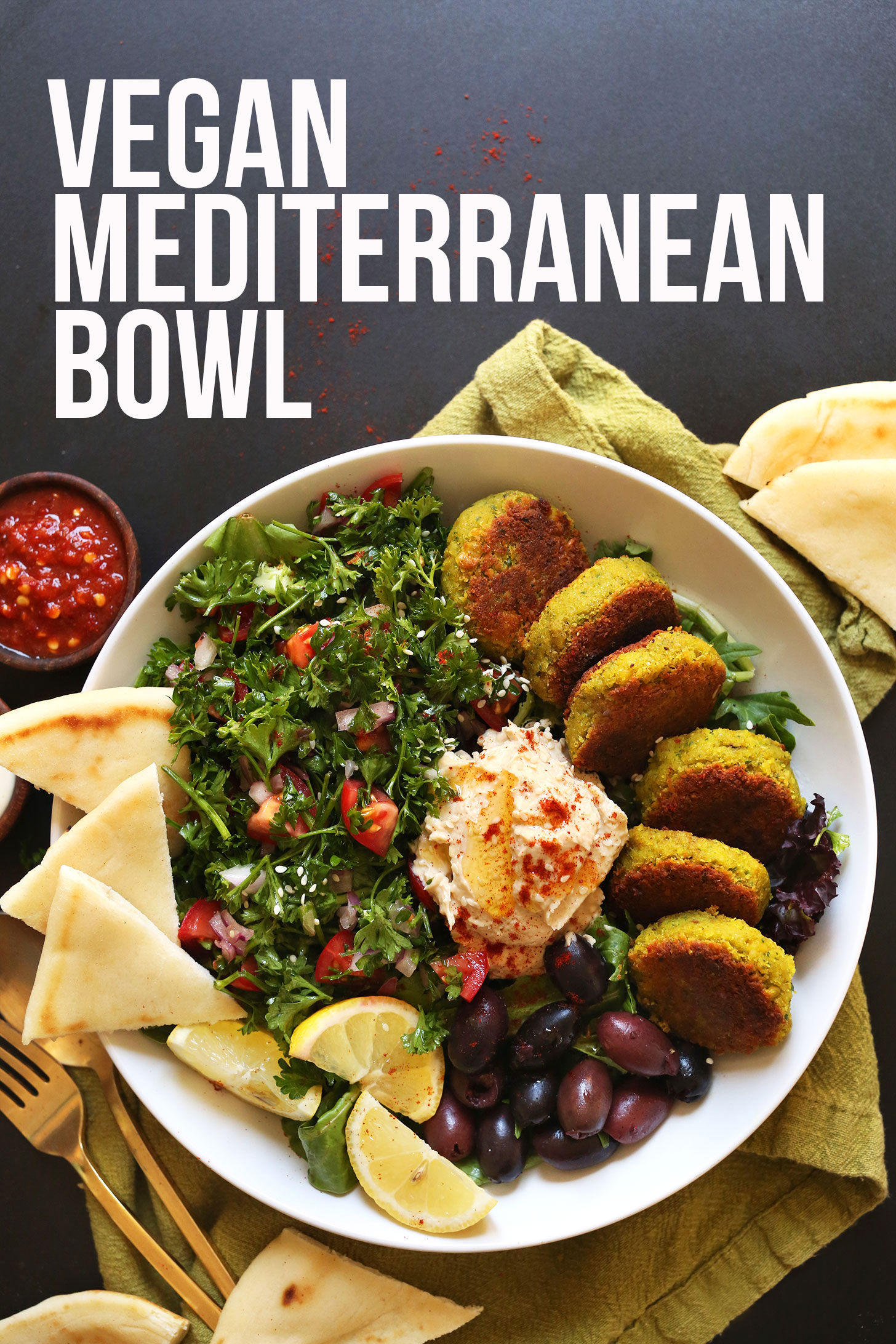This advertisement features a vibrant "Vegan Mediterranean Bowl," displayed against a dark gray background. The bowl, artfully arranged and showcased in the center, sits atop a green napkin. The well-balanced composition includes an array of colorful ingredients: lemon wedges, black olives, chopped tomato, and a mix of various vegetables in shades of purple, green, red, and orange. Pita bread pieces are both inside and outside the bowl, and scattered red pepper or hot sauce adds a touch of spice to the scene. A visually appealing aspect includes something fried, which could be a veggie cake or fried zucchini. Also present are triangular slices that could be cheese or another vegan substitute. Garnishing the dish is a tangy kale salad, adding a healthful crunch. The setting is completed with visible silverware, including forks and a spoon, adding to the inviting and artistic culinary presentation.